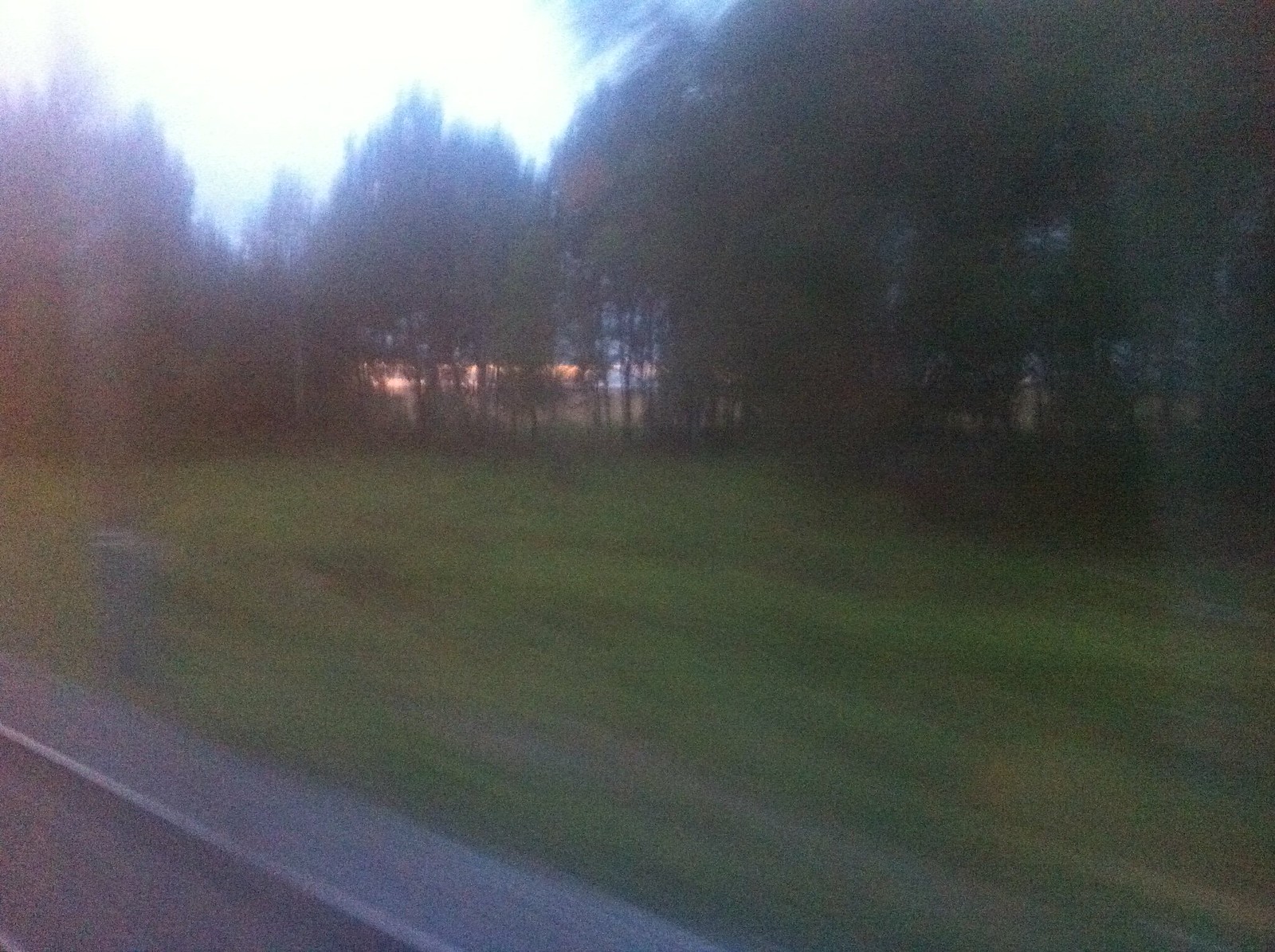This photograph captures the blurriness typical of an image taken from a moving vehicle. The scene is viewed from inside a car, partially showing a narrow sidewalk. The sidewalk is so slim that it seems it could only accommodate one person at a time. Alongside it, several posts are visible. The majority of the image consists of a flat green field, which stretches out towards the background filled with tall trees. These trees dominate the backdrop, with just a small glimpse of more flat land behind them. The image is bathed in the warm hues of sunset, with the sky near the horizon glowing in shades of orange and red, while the upper part of the sky retains a light blue tint.